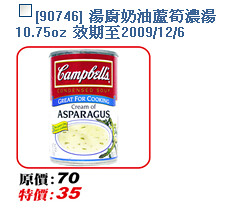This image depicts the front view of a can, prominently positioned at the center. In the top left corner, there is a small white square outlined in blue. Next to the square, the text "border 90746" is displayed to the right. Adjacent to this, blue Chinese characters are present. Below these characters, the text "10.75 oz" is printed. Further right, three additional Chinese characters are seen, followed by the date "2009-12-6". The can itself features the iconic "Campbell's" logo at the top, with the slogan "Great For Cooking" displayed beneath it.